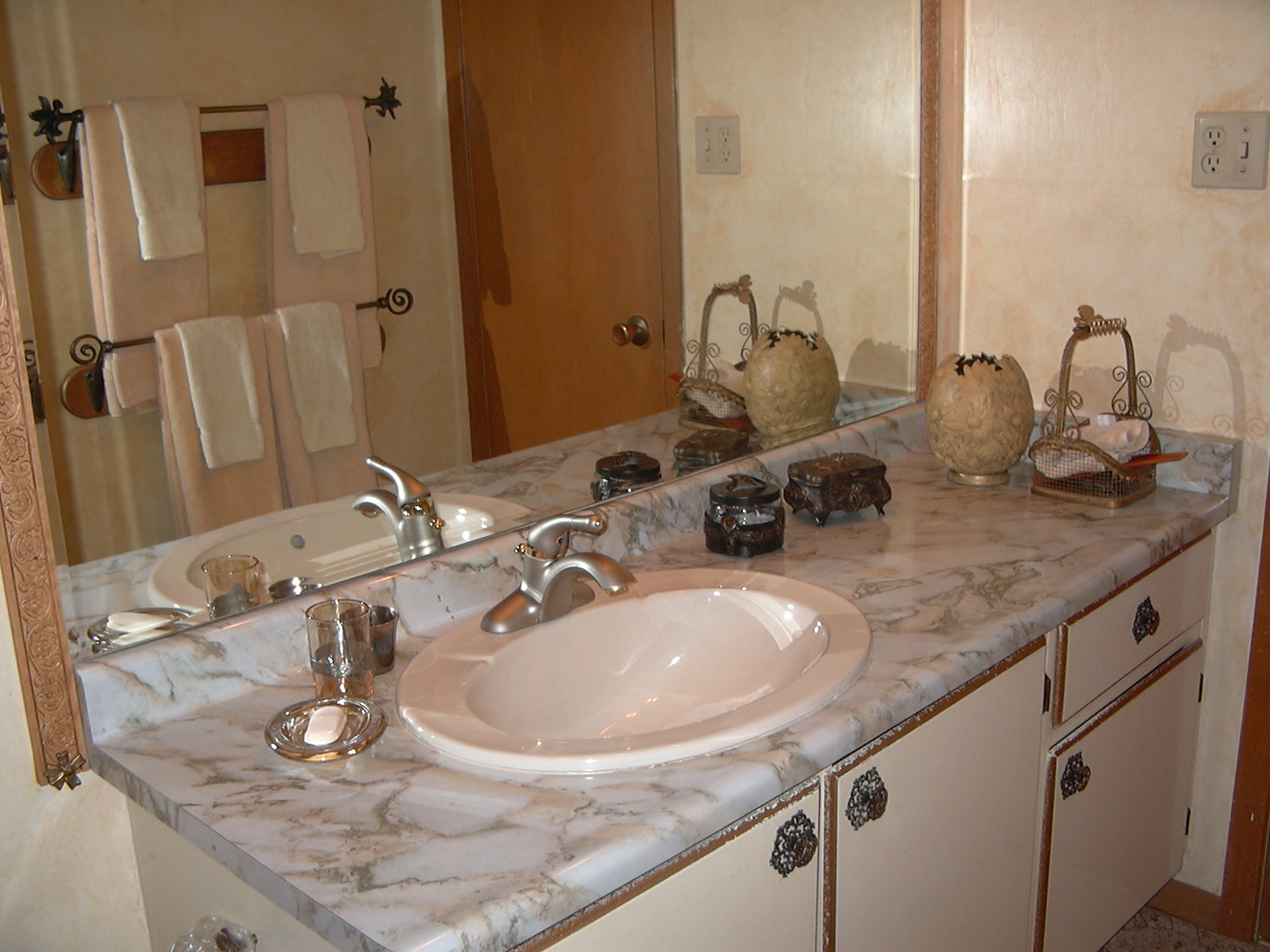This indoor photograph captures a meticulously detailed bathroom setting focused on a white sink, complemented by a silver faucet and accompanying water handle. The sink is integrated into a diagonally oriented, elongated rectangular countertop made of marble, featuring a subtle interplay of white and pink coloring. On the far end of the countertop, there is a wire basket along with a variety of items including a lighting fixture or vase, a compact metal box with short, small legs, a soap dish, and a glass cup.

The backdrop showcases a wide mirror that reflects a portion of the bathroom’s interior. Two towel bars affixed to a yellow wall are visible, each adorned with a neatly hung set of towels. The upper and lower towel bars both display a wide, long pink towel layered beneath a shorter white bath mat. These towel bars are mounted on a wooden bracket, adding an element of rustic charm to the decor.

Furthermore, the mirror captures the reflection of a brownish wooden door, accentuating the warm tones of the room. Directly beneath the sink, a white cabinet with a brown outline at its base provides functional storage while enhancing the aesthetic appeal of the space.